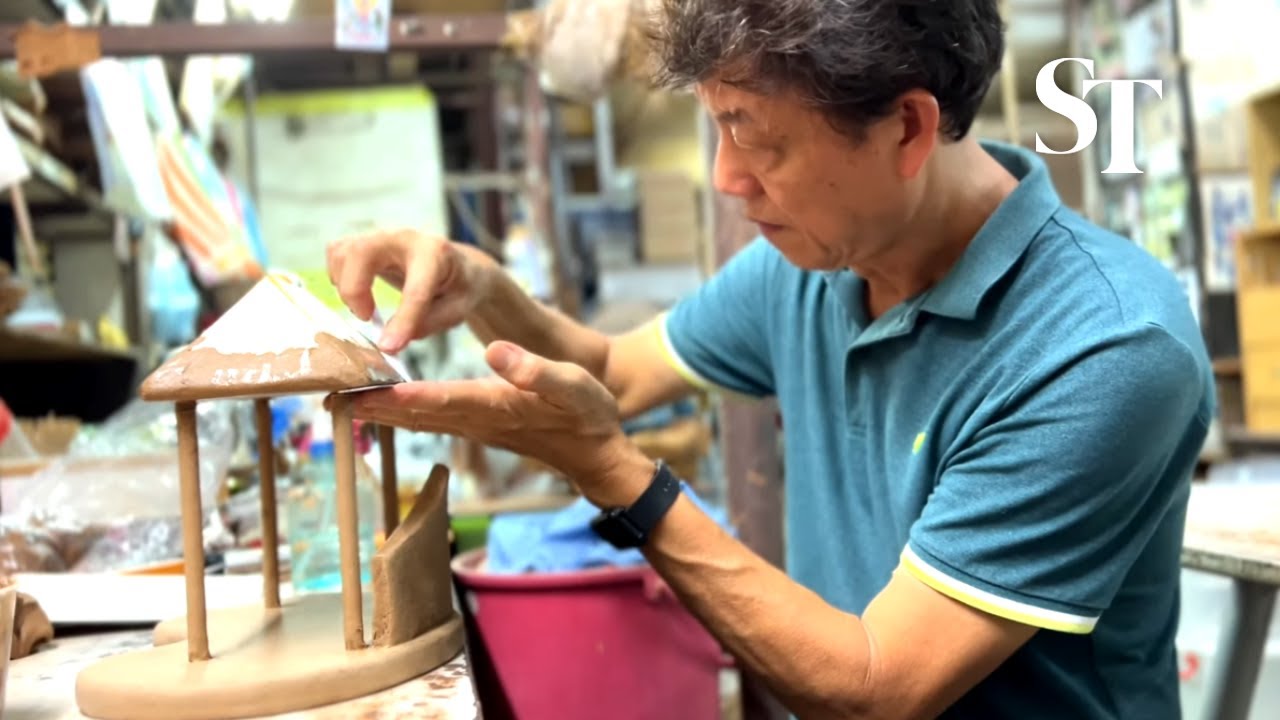In this detailed photograph, a Japanese artisan is captured meticulously sculpting the early stages of a small clay model resembling an open-sided hut or gazebo, characterized by four supporting posts and topped with a four-sided pyramidal roof. The artisan, wearing a blue short-sleeved collared polo shirt with yellow trim and a dark digital watch on his left wrist, is positioned on the right side of the frame, facing left. His focused expression reveals his dedication to the craft, as he delicately pinches the edges of the miniature structure, which features a slightly rounded base and a tan-colored wedge extending upward. The background, though blurry, hints at the creative clutter of a workshop, with a pink plastic bucket lined with a blue tarp or garbage bag visible near the center bottom of the image. Above the artisan and to the right, the capital letters "S" and "T" in white are prominently displayed, adding a unique element to the scene.